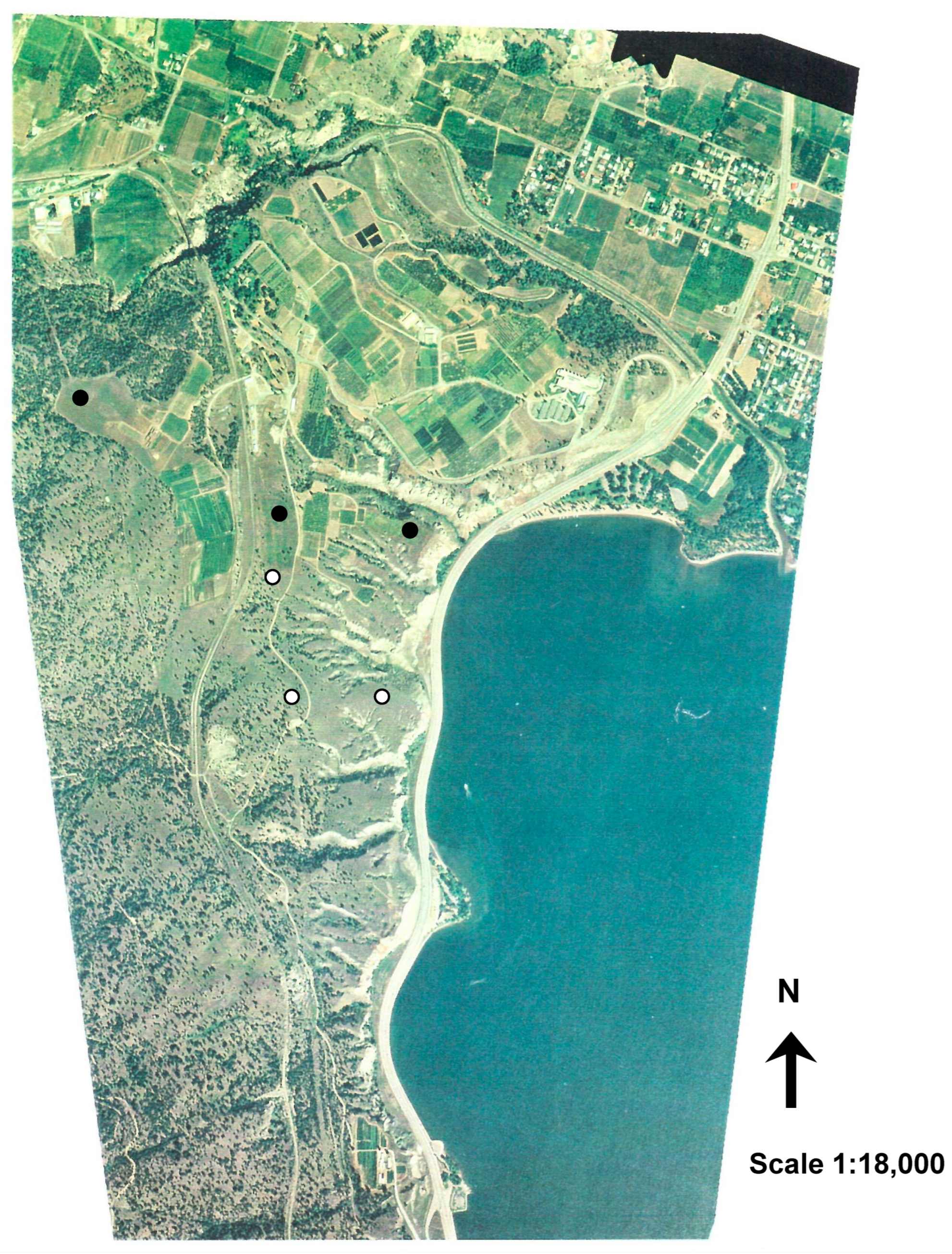This aerial image captures a striking overhead view of a small coastal town, presenting a vivid tapestry of land and water imbued with a greenish hue. The bottom right quadrant is dominated by a large water body, creating a serene backdrop against the plain, mostly unpopulated land to the left. The land is threaded with long, winding roads that appear like veins through the undulating terrain, likely mountains or hillsides. Above the water on the right side, a dense forest transitions into a cluster of white buildings arranged in both linear and horizontal patterns, suggesting an organized urban area. 

The left half of the image contrasts sharply, showcasing expansive farmlands or plains with minimal structural development, emphasizing the rural aspect of the landscape. Dotted across the map are various black and white markings, possibly indicating key points of interest or mapping coordinates. Near the bottom right corner, there is a small but essential legend featuring a compass pointing north and a scale of 1 to 18,000, providing a reference for the mapped area.

The entire scene, with its mosaic of shaded greens, pastel colors, and contrasting urban versus rural sections, strikingly resembles a detailed topographical map or even the intricately circuitous layout of a circuit board. This captivating aerial image is likely depicting a region along the east coast of America, evoking the landscapes typical of South Carolina with its beautifully parceled rural and urban expanses.